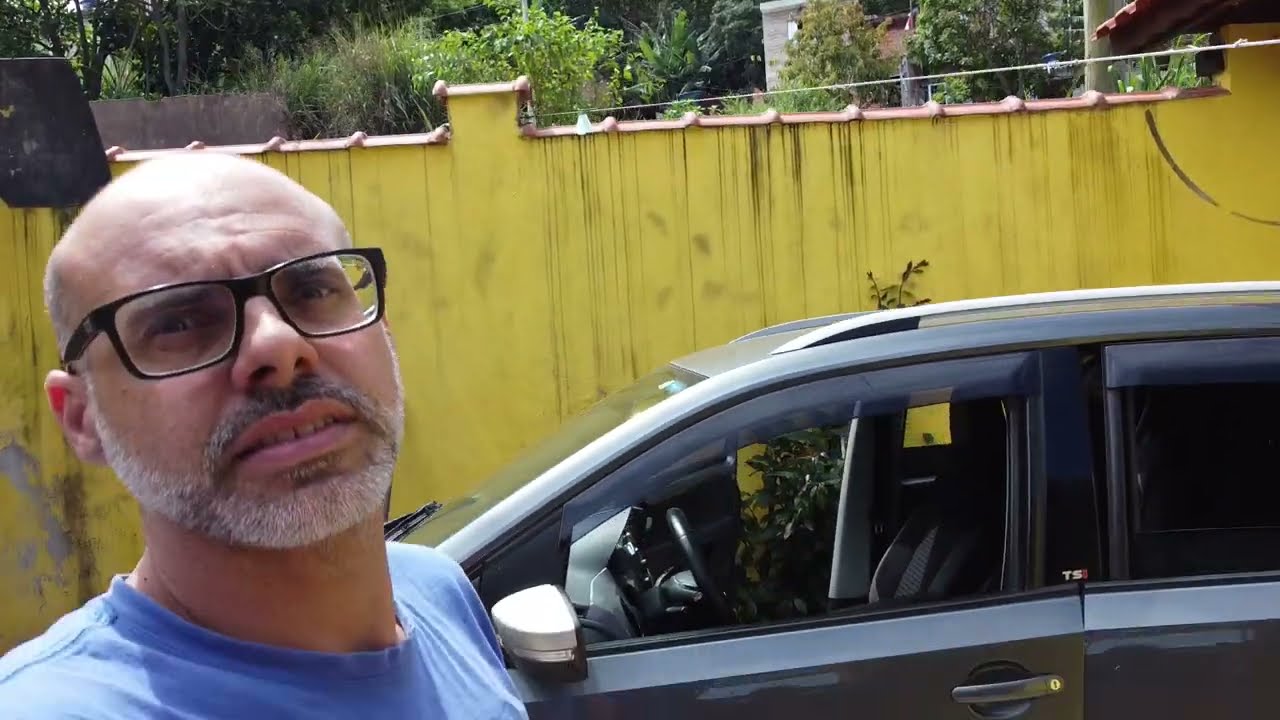A middle-aged, bald man with black-framed glasses and a distinctive handlebar white beard and mustache is taking a selfie from the left side of the frame. He is wearing a blue cotton t-shirt and has the slight grin of someone comfortably posing. The photo is taken in front of a dark grey SUV, whose passenger door is slightly ajar. The vehicle, which could be mistaken for a van due to its size and rooftop rack, has a black interior. In the background, a tall, approximately 15-foot high yellow wall stretches horizontally across the image, topped with red brick framing. Above the wall, the green leafy tops of trees are just visible. An electrical cord can also be seen running across the yellow wall. Some residential buildings peak from beyond the wall, adding layers to the scene's depth.